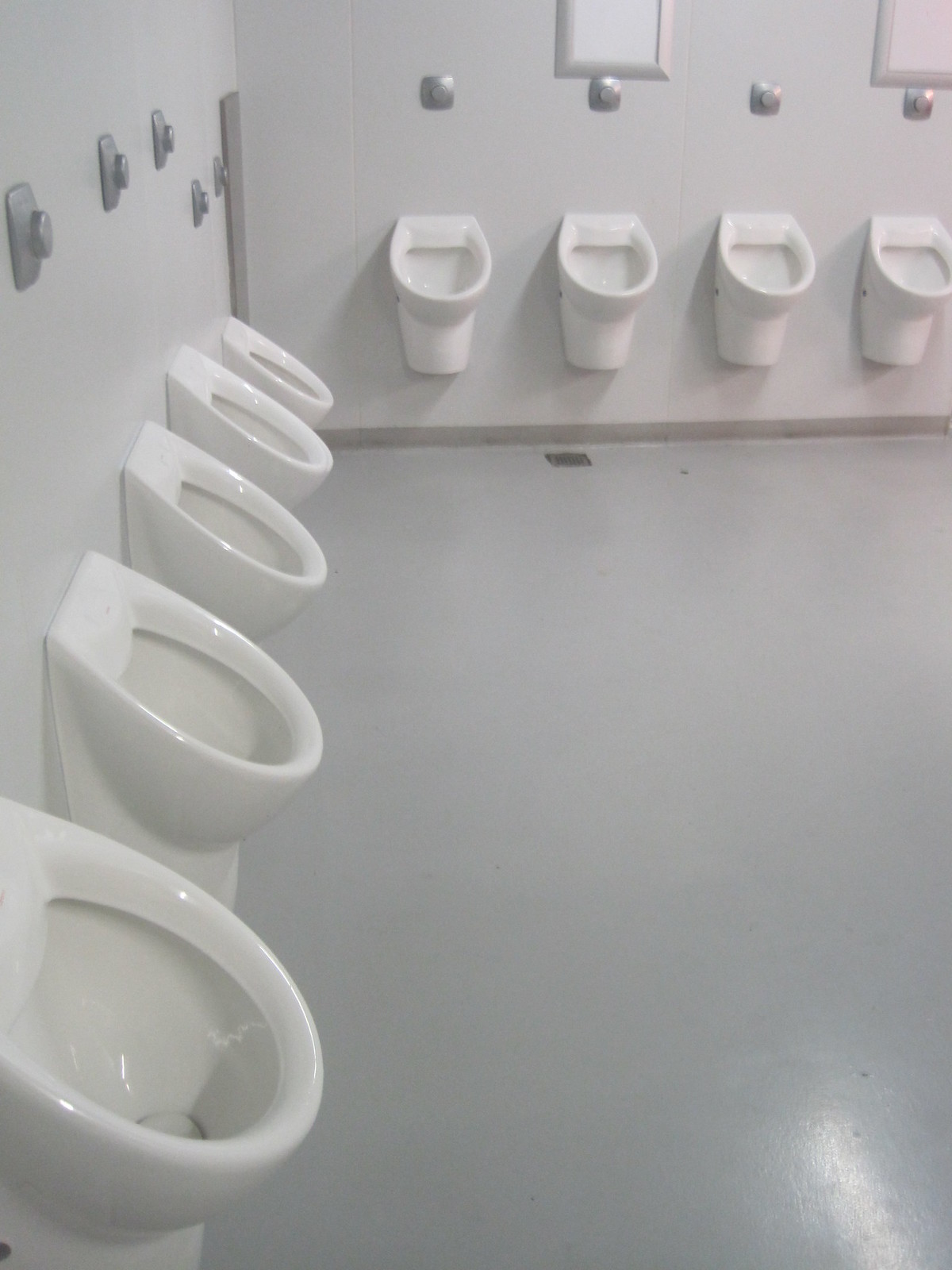This color photograph captures the interior of a men's bathroom, showcasing a total of nine white porcelain urinals arranged along two adjacent walls, viewed from an angle that places one wall on the left and another straight ahead. Each wall-mounted urinal is uniformly shaped and positioned a couple of feet off the smooth, light gray vinyl floor. The left wall features five urinals while the wall ahead displays four more, creating a right-angle layout in the corner of the room. The urinals are accompanied by silver flush buttons at a convenient height for standing users. The surrounding walls are painted in cream to complement the flooring. Additionally, the wall in front includes two posters, though their contents are indiscernible.